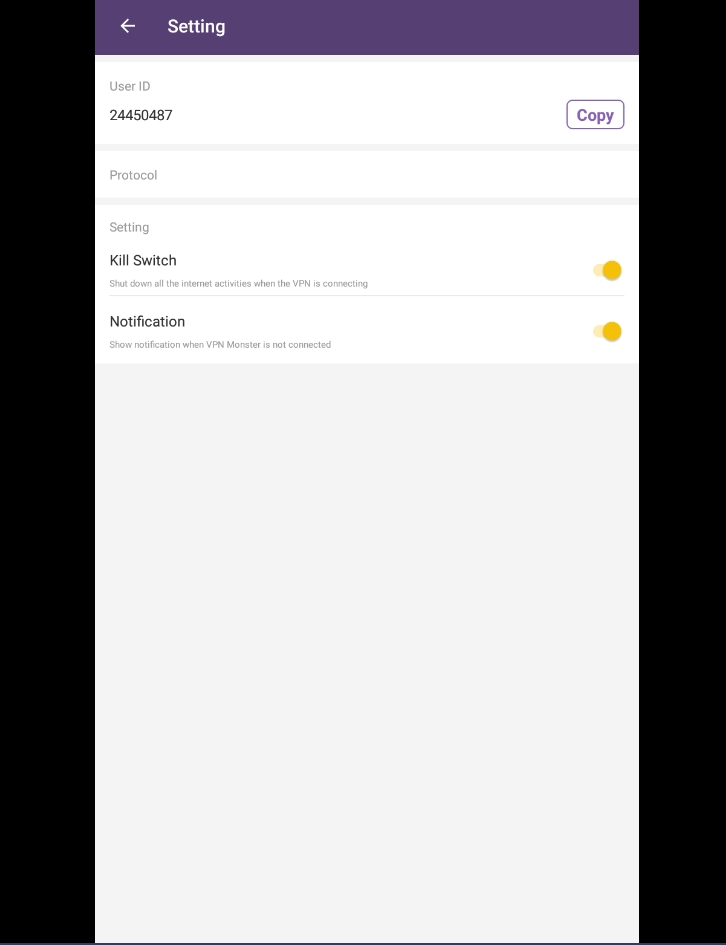Screenshot of a settings page on a mobile device. The image is framed by two thick black borders on the left and right sides. At the top, a purple header features a back arrow and white text that reads "Settings." Below the header, "User ID" is displayed in small gray text with the ID number "24450487" in black font underneath. To the right of the ID, a white button with a thin blue-purple border and purple text allows users to "Copy" the ID.

Further down, "Protocol" is labeled in small gray text but is currently empty. In larger black text, the setting "Kill Switch" is shown with a yellow toggle button on the right, indicating it is turned on. A subtext explains, "Shut down all internet activities when the VPN is connecting." 

Following a dividing line, the setting "Notification" is displayed in the same larger black font. Underneath, it says in smaller gray text, "Show notification when VPN monster is not connected," with another yellow toggle bar on the right, also in the on position.